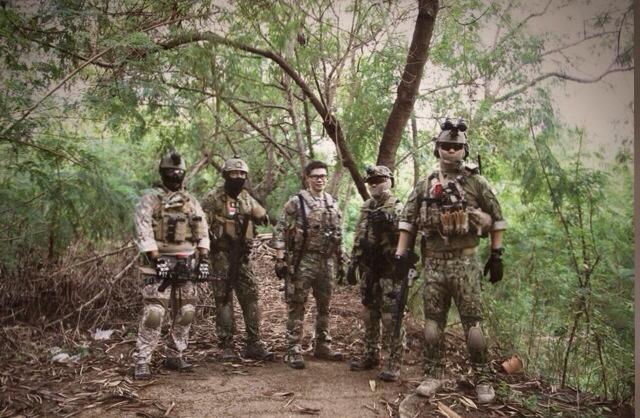The photograph is rectangular and taken outdoors in a dense, jungle-like area, featuring a small clearing surrounded by lush greenery, trees, and overhanging shrubs. The ground is covered in dirt, dried leaves, and twigs. In this setting, five men stand in a semicircle, posing for the shot. They are all donned in full military gear, including fatigues with varied camouflage patterns like olive and brown that blend seamlessly into the forest background. The men are equipped with artillery vests and black gloves, most have their sleeves partially rolled up. Several are masked, obscuring the lower half of their faces, and some wear sunglasses and helmets. One soldier, standing to the right, is dressed in a khaki uniform, brown boots, and features several small flashlight devices on his head. He carries what appears to be either canteens or additional weapons on his chest. Another soldier on the far left holds an automatic gun with both hands. Only the man in the center is helmetless and instead wears glasses. Despite the inability to see their full expressions clearly, they exude a masculine and imposing presence, likely suggesting they are a revolutionary force or a guard force in a tactical, forested setting.